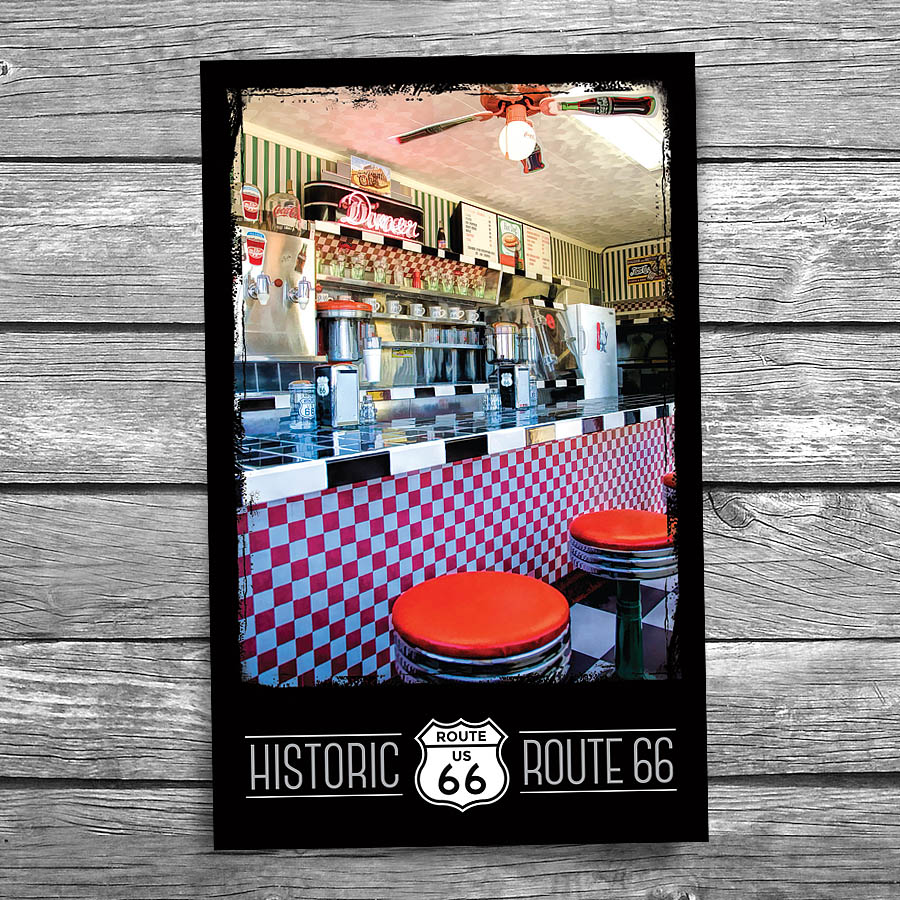The image depicts an advertisement poster for a historic Route 66 diner, affixed to a wall with gray, weathered wooden planks. Central to the poster is a classic 1950s-style diner scene dominated by a red and white checkered theme. The diner’s counter is adorned with red and white checks, topped with a black and white checkered surface. Several red bar stools, with two prominently in view and a partial third stool just visible, line the bar. Behind the counter, a collection of stainless steel appliances is neatly arranged, including a soda fountain machine with Coca-Cola advertisements, coffee machines, and a small white refrigerator. Shelving above the counter holds glasses, and a bright neon sign spells out "Diner." The bottom of the poster features the iconic "Historic Route 66" insignia, tying the nostalgic ambiance to the famous American highway.